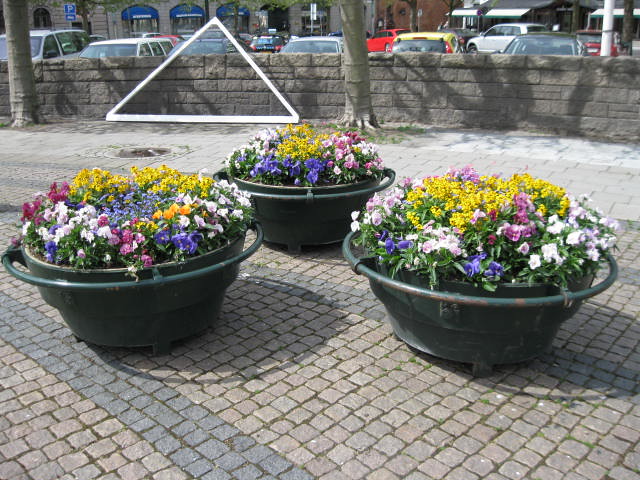The image shows a vibrant commercial area with a cobblestone street composed of light and dark gray bricks. Dominating the foreground are three massive, round, and intricately designed flower pots, each about five feet in circumference. The pots appear to be made of painted metal and come in shades of pale green and dark gray. They hold an array of colorful flowers—white, purple, pink, yellow—set against a backdrop of lush green leaves. Centered on the sidewalk, these decorative pots form a triangular arrangement.

Beyond the flower pots stands a gray stone retaining wall, separating the sidewalk from a parking lot where various cars are parked—gray, white, red, black, and yellow vehicles can be seen. Flanking the wall to the left are two tree trunks, which are partially obscured, and between them is a white triangle shape that could either be a structure or a car’s windshield. In the further distance, a commercial shopping area can be seen with buildings, some adorned with blue awnings.